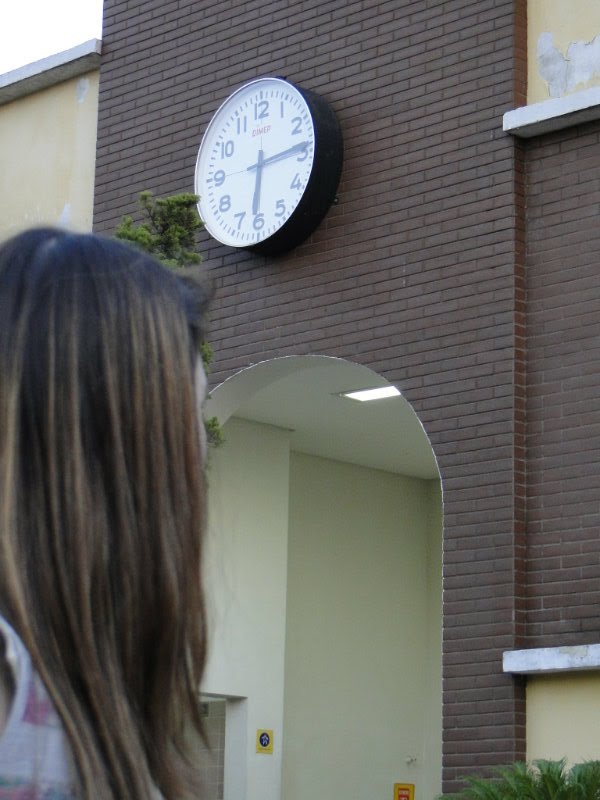This photograph captures a visually engaging scene of a building with a brick façade, featuring a prominent arched opening. Above the archway, a large, circular clock with a white face and black numerals, reminiscent of a standard school clock, displays the time 6:14. In the foreground, on the bottom left, stands a woman with long brown hair, turning her head upwards towards the clock. Her partial profile and the detail of her hair are visible. The archway provides a glimpse into the building's interior with white walls and what appears to be the outline of an elevator. Near the left side of the archway is a tall tree, partly obscured by the woman's head. The right side of the archway is bordered by dense shrubbery, adding a touch of greenery to the scene.